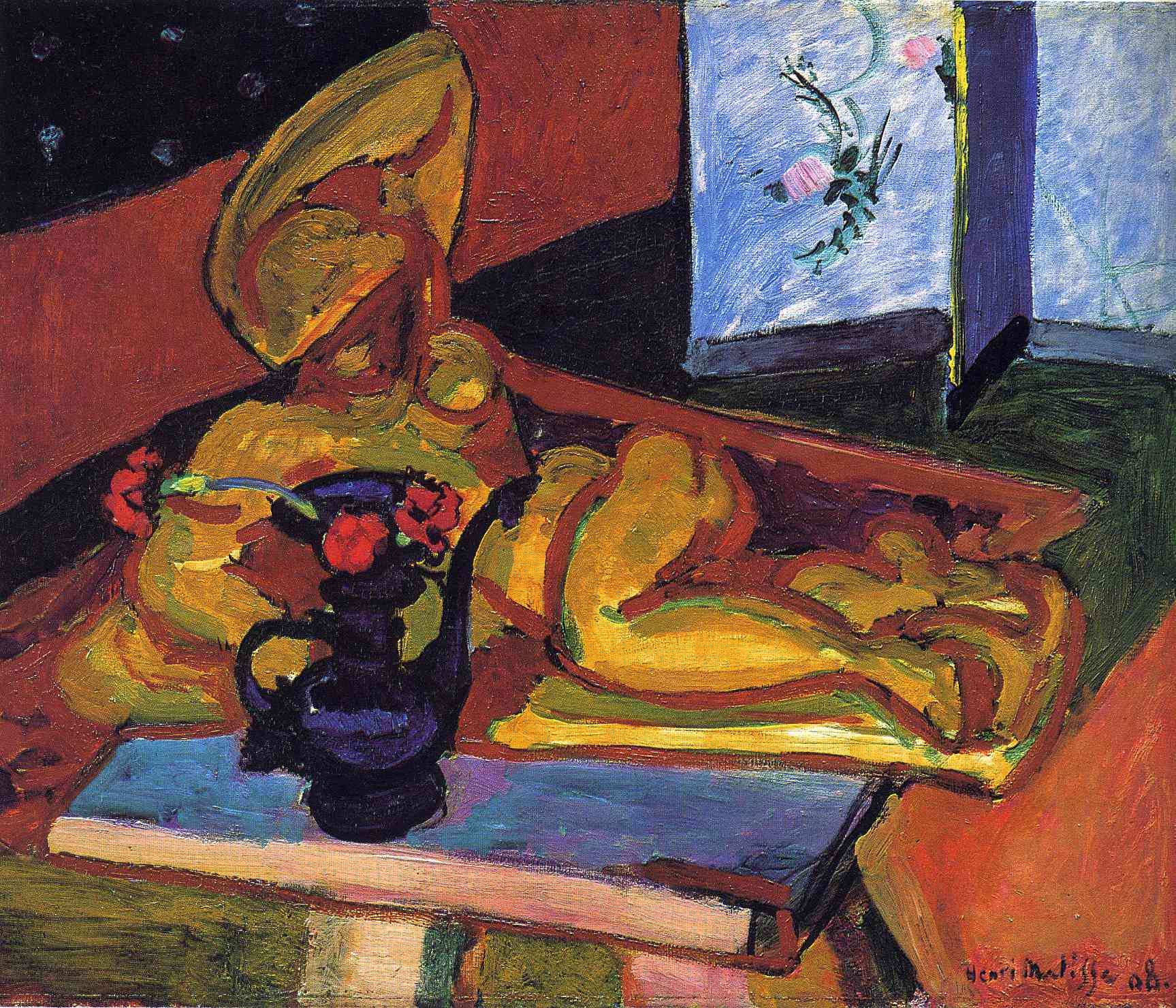The image is an abstract painting featuring a central figure depicted in gold and mustard yellow tones with a reddish-maroon outline. The person is lying on their right side with their left leg draped over the right, and their torso twisted upwards. They have their left arm bent and resting on their head while their right arm supports them. The background includes a blue wall adorned with green vines and pink flowers in the upper right corner. A low blue table sits in the foreground, holding a black vase filled with red flowers and green stems. The upper left corner features a black sky with white dots resembling stars, while the left side of the painting shows a red wall. The painting is rendered in bold, rough brushstrokes, emphasizing the vibrant and dynamic color palette. The artist's signature, potentially reading "H-C-A-R-I-M-A-L-I-S-S-E 08," is located in the lower right corner. The overall composition is filled with rich colors, including patches of blue, orange, and green, creating a vivid and striking visual impact.